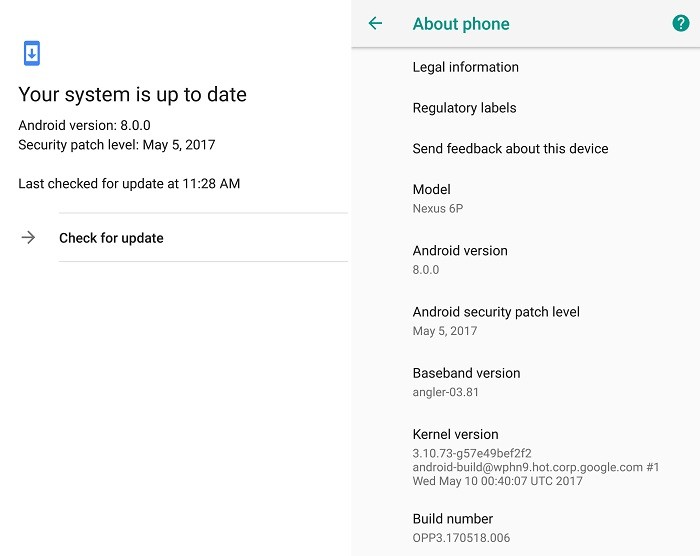The image depicts the settings screen of a smartphone, specifically focusing on the device's software information. The top portion of the screen displays a logo featuring a phone with a downward arrow, accompanied by the message "Your system is up to date." The Android version is 8.0.0, with the security patch level dated May 5th, 2017. The last update check was conducted at 11:28 AM, and there's an option to "Check for update" indicated by an arrow.

A pop-up overlay provides additional details about the phone. An arrow at the top allows users to navigate back to the previous screen. In the upper-right corner, a green circle with a check mark signifies that the device is current with all updates. Below this, several options are listed:

1. **Legal information**
2. **Regulatory labels**
3. **Send feedback about this device**

Further information about the device includes:
- **Model:** Nexus 6P
- **Android version:** 8.0.0
- **Android security patch level:** May 5th, 2017
- **Baseband version:** Angular.03.81
- **Build number:** 0PP3.1.70518.006
- **Kernel version:** 3.10.73-g57e49bef2f2, with a note of "Android-build@WPBN9.hot.corp.google.com #1" and the date Wednesday, May 10th, UTC 2017.

This detailed screen provides comprehensive information on the device's software status and version history.